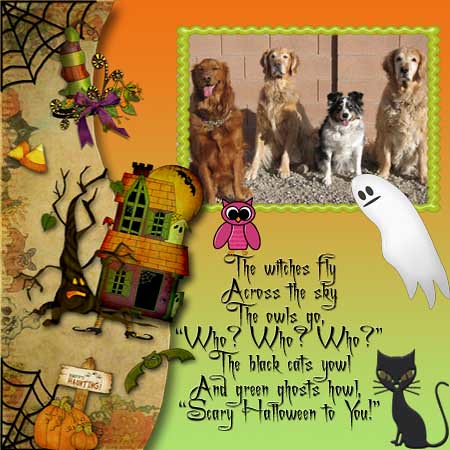This Halloween-themed image resembles a scene from a children's storybook. Dominated by vibrant lime green and orange hues, its center features intricate, playful graphics. At the very top, nestled in a squiggly yellow frame against a gray concrete background, a photograph showcases four dogs: a Labrador Retriever on the left, another lighter-colored Labrador next to it, followed by a smaller black and white Border Collie, and a fourth dog, possibly an English Sheepdog. Below this photo, scattered across the scene, are cartoonish elements — a ghost and a cat drawing, a pink owl with black eyes, spiderwebs, candy corn, and a scary haunted house with bare-branched trees, one of which has a face with yellow eyes and an open mouth. The right center of the image displays a playful pink owl, and the bottom right corner features a black cat with green eyes and whiskers staring directly at us. The text in special Halloween print reads, "The witches fly across the sky, the owls go hoo, hoo, hoo. The black cats yowl and green ghosts howl, scary Halloween to you."